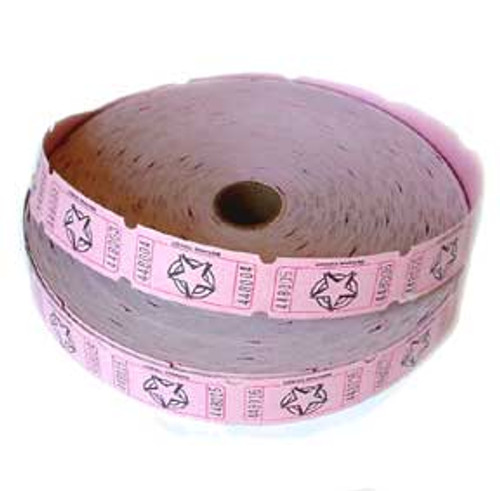A vibrant pink roll of brand-new arcade tickets, meticulously wound into a thick cylinder, dominates the image. Each ticket features a prominent black star centered within a bullseye-like design, comprised of two concentric circles. Numbers are printed on both the left and right sides of each ticket, though they are somewhat hard to read; one ticket near the top center prominently displays "448604," while the next ticket ends in a 5. The roll, approximately six inches in diameter, has an unused, pristine appearance, with its perforated edges neatly aligned aside from a single ticket peeling slightly upwards. The roll is positioned against a black background, emphasizing its vibrant color and detailed design, including a cardboard ring at the center meant to facilitate easy dispensing.